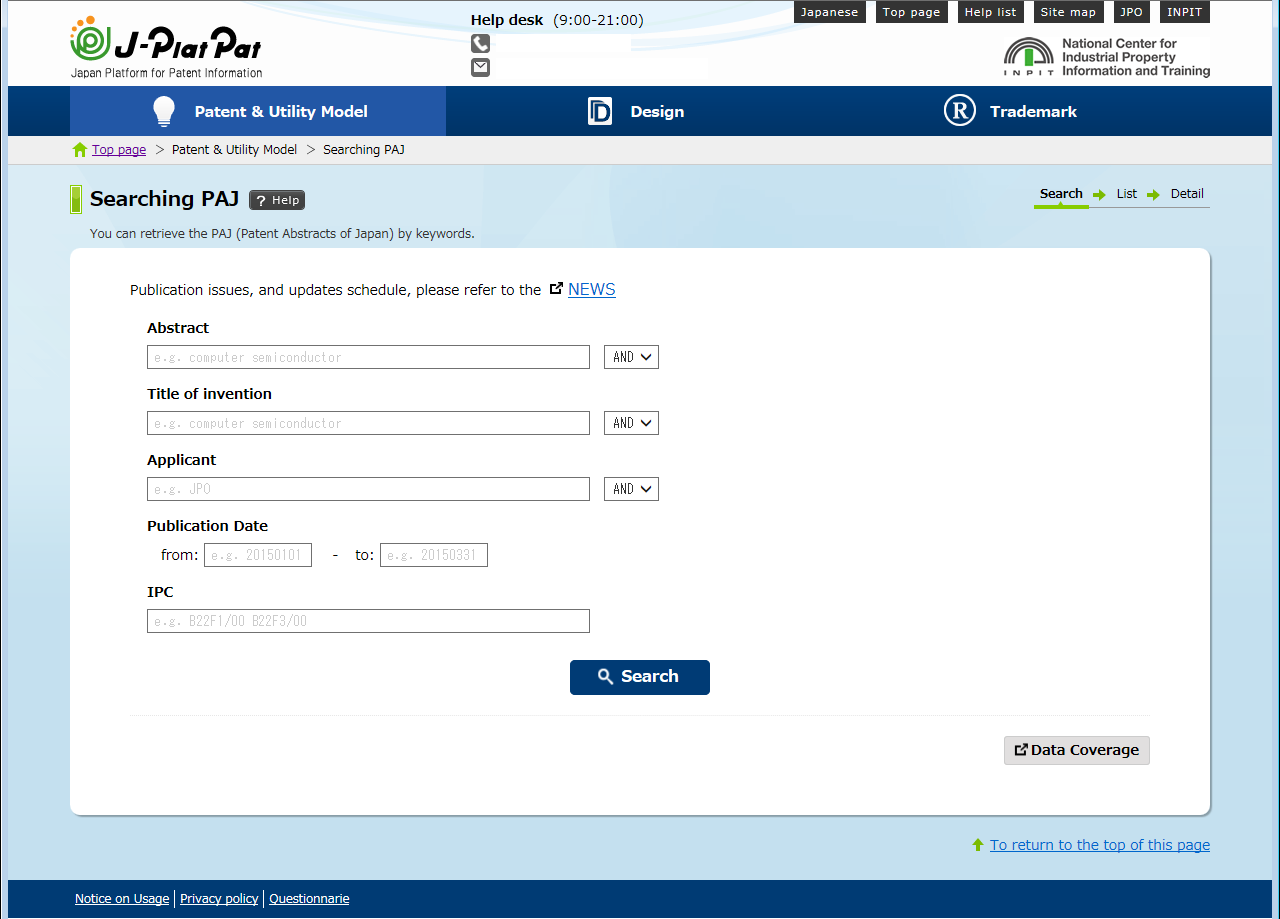Screenshot of a web page displayed on a laptop or monitor with a light blue background. The top of the page has a white background with a logo in the top left corner resembling a stylized "P" and "J" in a spiral shape, colored green with small orange dots above it. The company name "J-PLAT PAT" is displayed next to the logo, though the text beneath it is unreadable. Centrally located at the top of the page, it states "Helpdesk 9 to 2100 hours" with accompanying icons for phone and email.

There are six black tabs below this information, some of which are labeled "Sitemap" and "Input," but the rest are not clear. Below these tabs on the white bar is the text "National Center for Industrial Property Information and Training" with a logo that resembles an archway.

A blue horizontal bar spans the screen with menu options labeled "Patent and Utility Model" (accompanied by a light bulb icon), "Design" (with an icon of a white square containing the letter "D"), and "Trademark" (with an "R" inside a circle indicating a registered trademark). The "Patent and Utility Model" option is highlighted in a lighter blue, indicating it is currently selected.

The majority of the light blue background is occupied by a large white rectangular section titled "Searching P.A.J." The text explains that you can retrieve "Patent Abstracts of Japan" by keywords. This section includes dropdown menus labeled "Abstract," "Title of Invention," and "Applicant," each with a drop-down arrow and potentially an auto-fill feature. Below these menus, there's an option to filter by "Publication Date" with fields to input start and end dates. A prominent blue "Search" button is located at the bottom of this white rectangle.

Below the rectangle, on the light blue background, there's a blue hyperlink reading "To return to the top of this page, click there," accompanied by a green upward-pointing arrow.